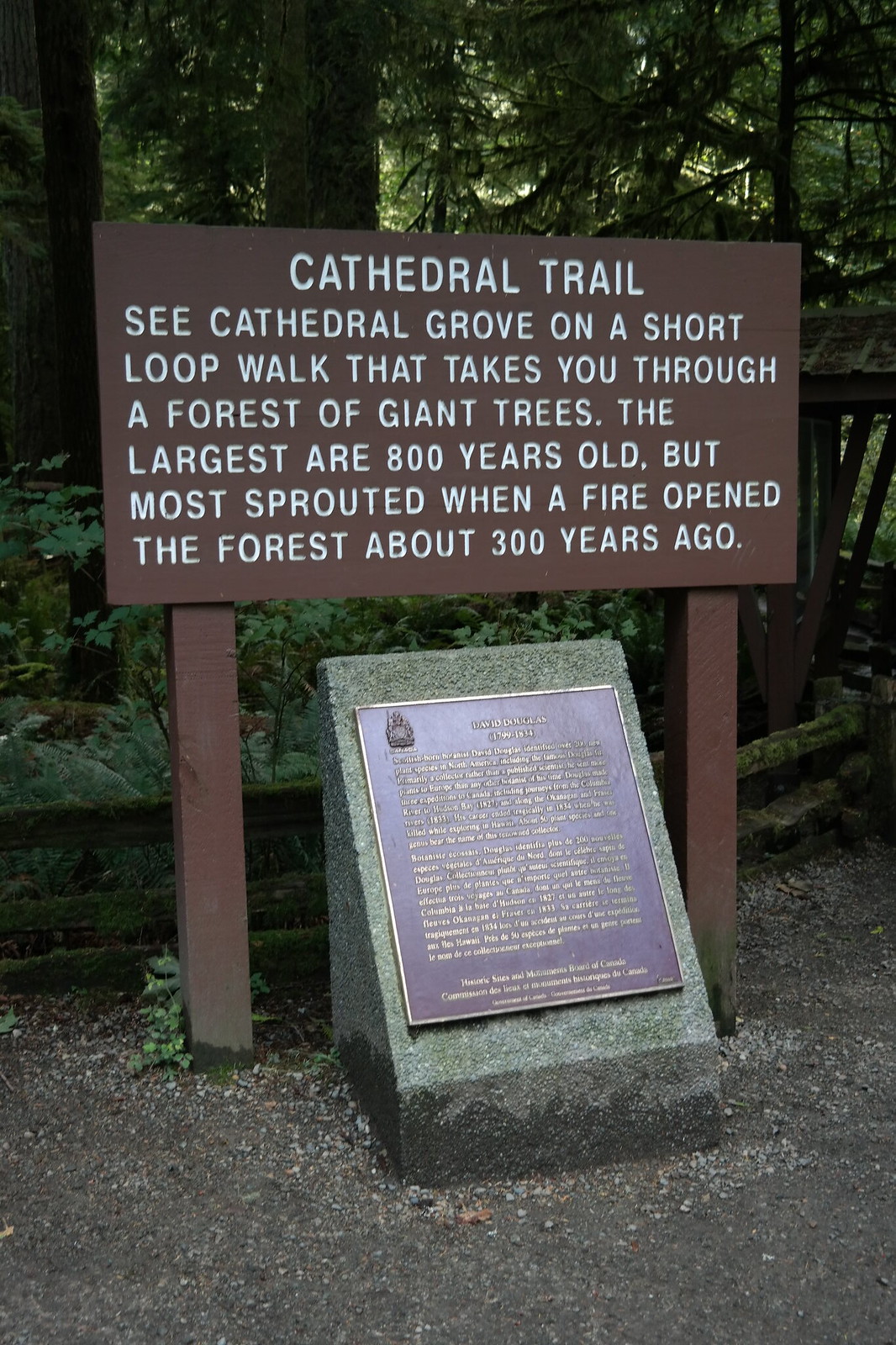The photo captures a picturesque scene taken outdoors featuring two prominent signs set against a lush backdrop of trees, bushes, and greenery. At the forefront, there is a gravel or asphalt walkway leading up to the signs. The main wooden sign is mounted on two wooden posts and painted brown with white lettering that reads: "Cathedral Trail. See Cathedral Grove on a short loop walk that takes you through a forest of giant trees. The largest are 800 years old, but most sprouted when a fire opened the forest about 300 years ago." Below this wooden sign, embedded in a concrete or stone base, is a bronze plaque with unreadable text. A variety of foliage, including shrubs, accentuates the natural beauty surrounding the sign, indicating that this is likely a trailhead within a park or nature reserve.